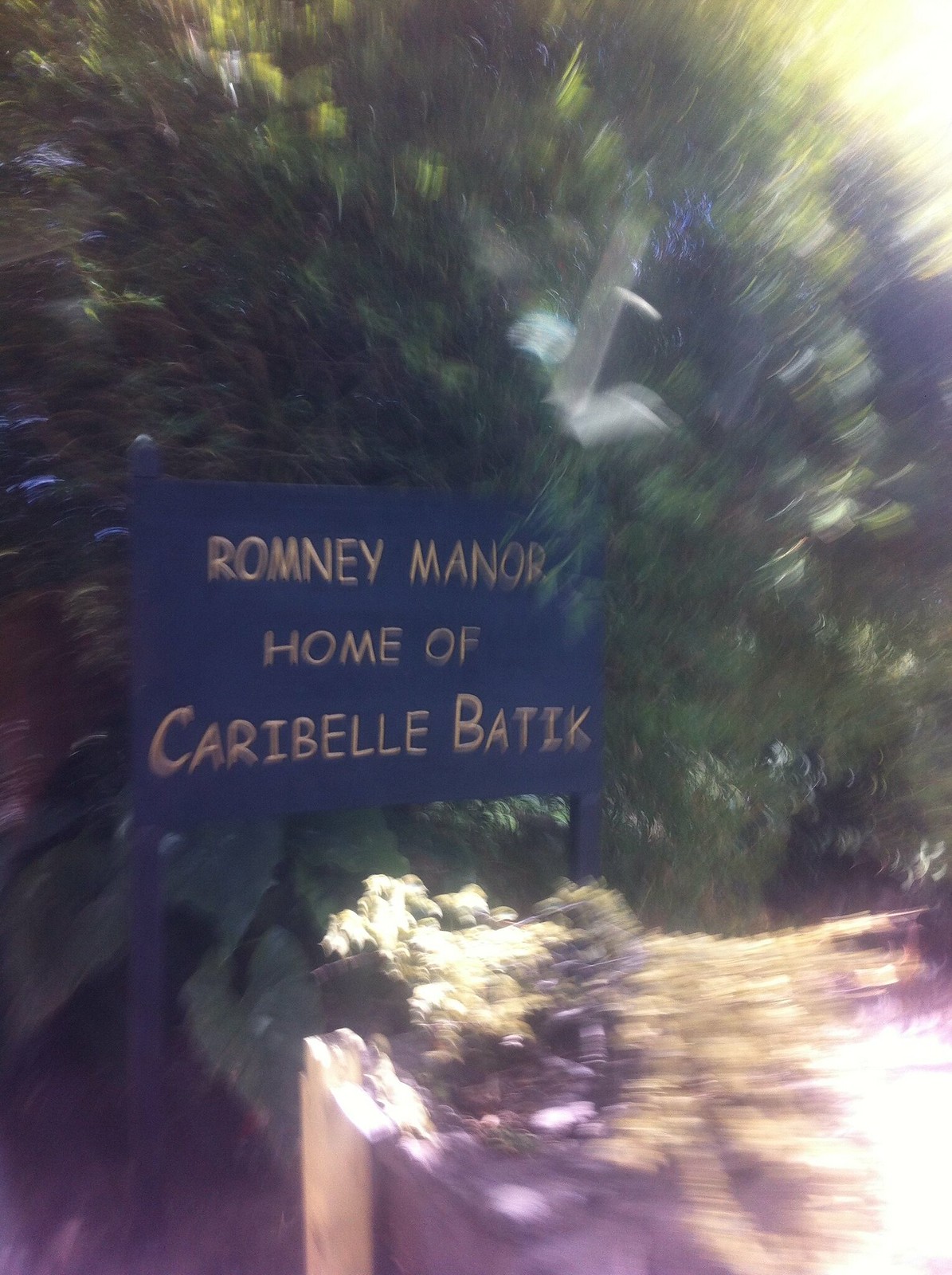Outdoor daytime photograph taken in bright light with a focus slightly left of center. The central feature is a rectangular blue sign with yellow lettering. At the top, it reads "Romney Manor," followed by "Home of," and at the bottom, "Caribelle Batik." The background is filled with lush green trees that extend to the edges of the frame and occupy the upper left and right corners. To the right, there is a visible path or trail starting at the lower right edge and curving out of the frame. A wooden post is partially visible just left of the foreground center. The light source is coming from the upper right, brightening the lower right corner. The entire image is notably out of focus, indicating motion blur from the camera when the photograph was taken.